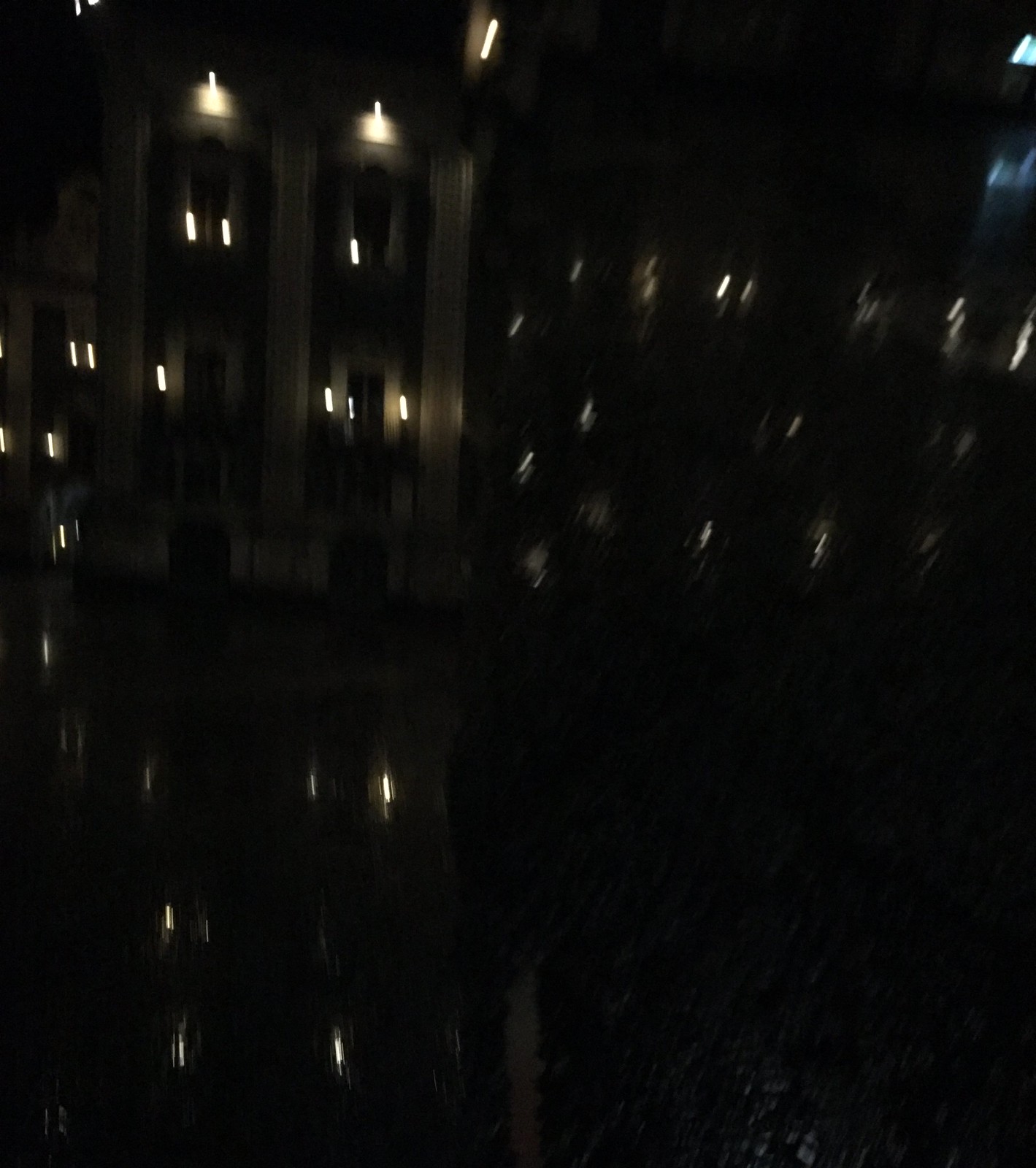The photograph depicts a tall, white, Art Deco-style building captured at night. Dominating the scene is the building on the left, with its distinctive vertical columns and rectangular windows that feature pillar-like or shutter-type structures along the sides. Above these windows is an arched segment with rounded lights on top, casting a subtle glow in the otherwise dark surroundings. 

In front of this building, there appears to be a reflective water surface, as the light patterns from the building are mirrored below, suggesting water is present. To the right of the image, there is a considerable dark mass, likely a tree or dense bushes, partially obscuring the view and lacking a clear reflection in the water, indicating the vegetation could be blocking the water's surface directly beneath it. 

Additional slanted lights suggest the camera might have been in motion during the shot. The setting is evidently a moonless night, making the scene challenging to interpret due to its overall darkness, with almost everything else in the image enveloped in black.